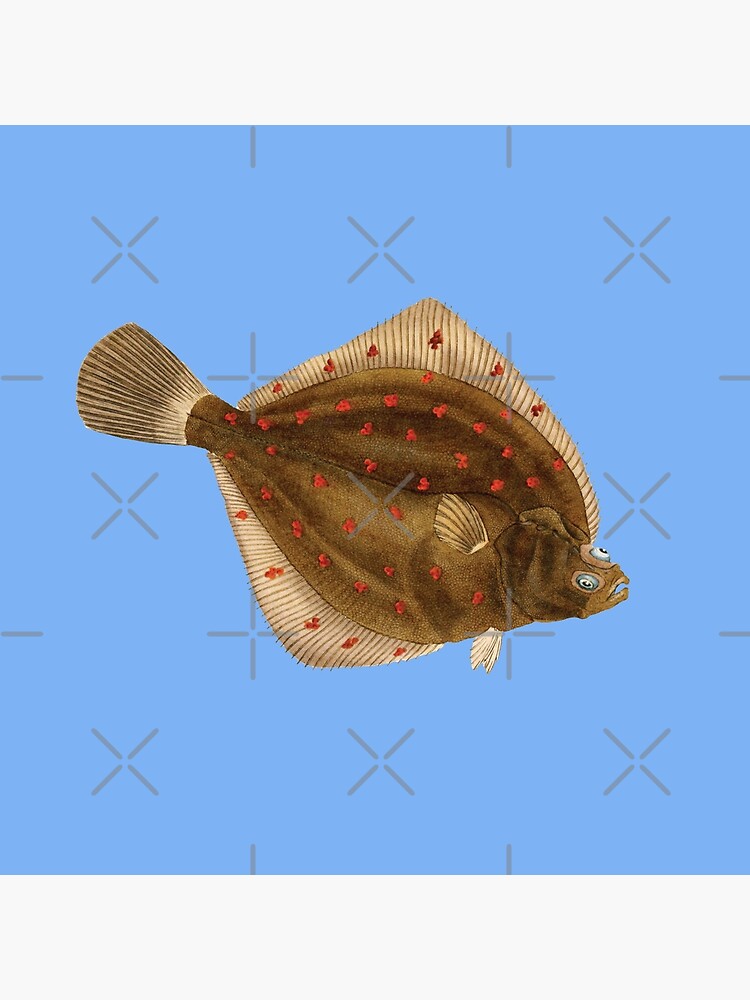The image showcases a detailed drawing of a flounder, centrally positioned on a light blue square canvas. The background is adorned with alternating rows of gray X shapes and plus signs, organized in a detailed pattern that adds texture to the scene. The flounder itself has a distinct oval shape and features a predominantly brown body adorned with numerous red spots. Its fins, including the tail, are a lighter tan or beige with fine lines, and it has a row of fins running along both the top and bottom curves of its body. The flounder's two blue eyes are uniquely placed, one on the side and one on top of its head. The small mouth is visible at the front, adding to the overall lifelike quality of the illustration. The intricate design choices and vibrant details, such as the contrast between the brown body and the blue eyes, make the artwork both striking and highly descriptive.